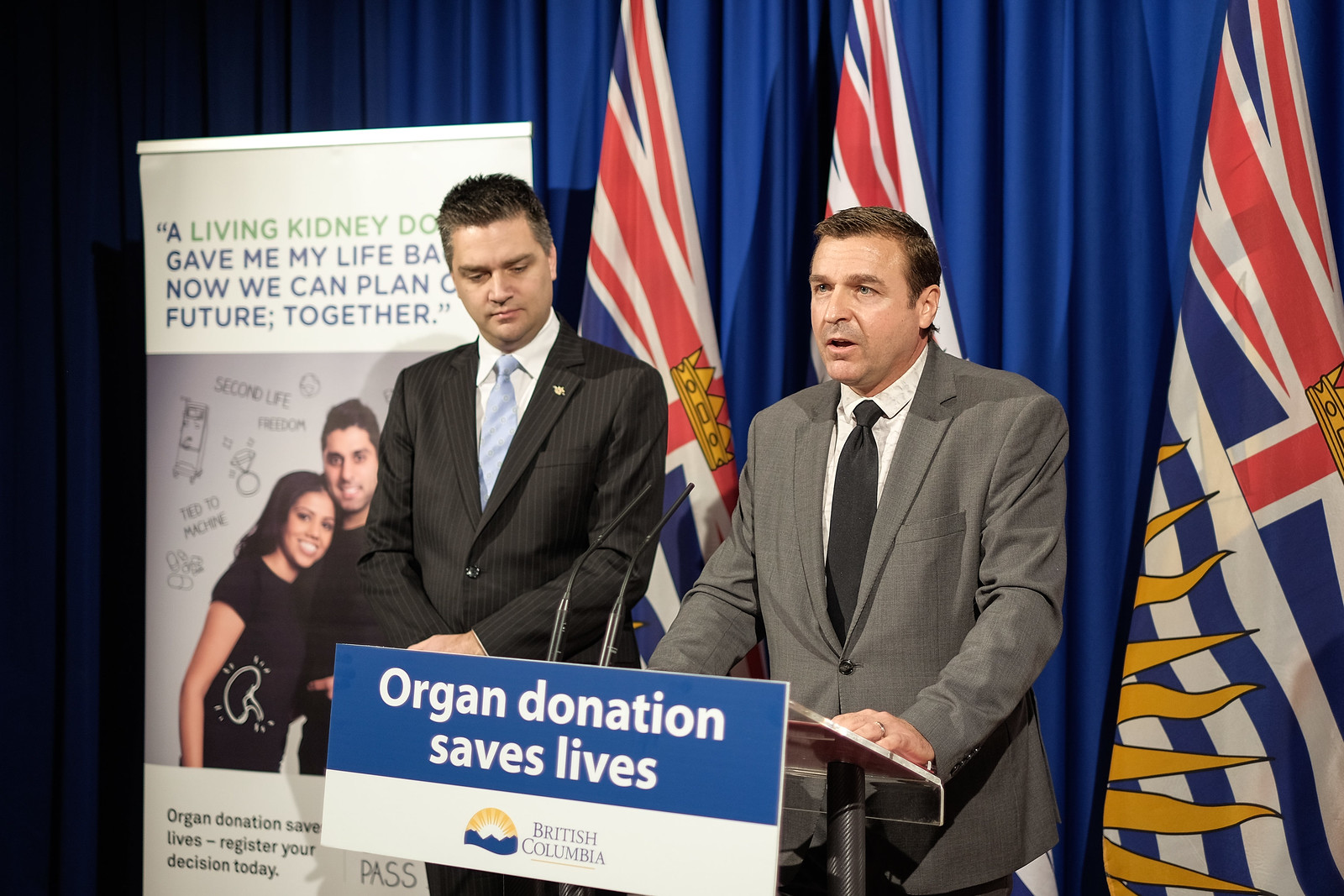This photograph captures an indoor presentation or conference room setting, showcasing a significant moment centered around the theme of organ donation. Standing at the podium, a white man dressed in a gray suit, gray tie, and white shirt addresses the crowd. The podium is marked by a sign that reads, "Organ Donation Saves Lives," accompanied by a logo depicting a blue mountain with a sunrise, representing British Columbia.

Next to the speaker, another white man in a gray suit and light blue tie, with his head bowed, listens attentively. To the left, a prominently displayed banner partially reads, "A Living Kidney Gave My Life Back, Now We Can Plan Our Future Together." The word "donor" and "back" are partially obscured by the speaker's head. The banner also features a photo of a white man and woman, both dressed in black, with the woman’s shirt displaying a graphic of a kidney. Below this image, the banner reiterates, "Organ Donation Saves Lives, Register Your Decision Today."

Behind the two men hangs a blue curtain, flanked by two flags; their red, white, and blue colors suggest they might be Union Jack flags, possibly representing New Zealand. Additionally, a portion of a flag presumed to be British Columbia's is visible, characterized by yellow sun rays and blue and white stripes, underscoring the regional context of this impactful event.